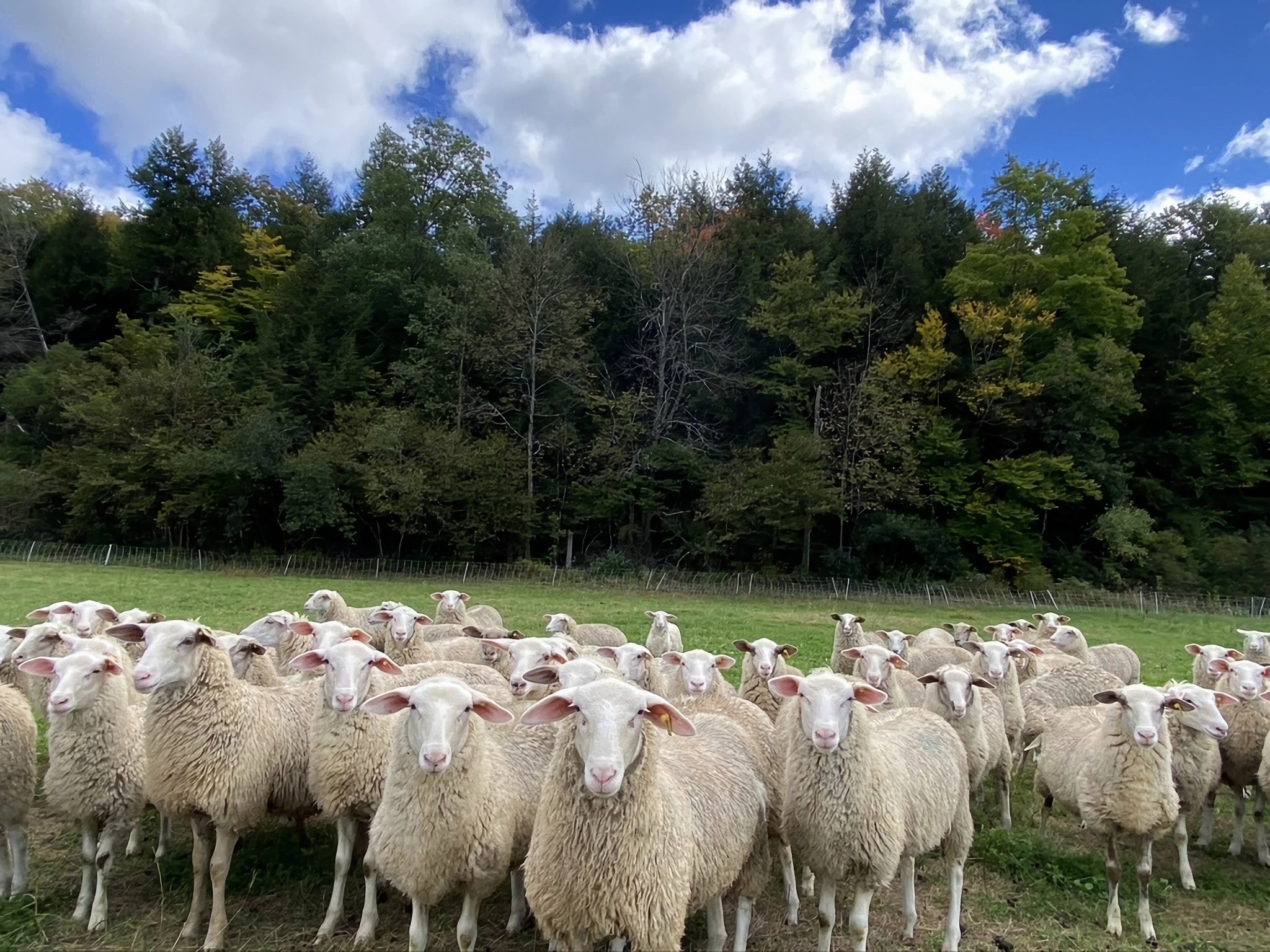This photograph captures an outdoor scene with a considerable flock of sheep gathered closely together, all facing the camera. The sheep have recently sheared, with mostly short, slightly off-white, wool and very white heads. They populate the entire foreground of the image, standing amidst a lush green pasture. Behind the sheep, a low, possibly chain-link or welded wire fence stretches across the photo's width, though its posts lean slightly. Beyond this fence lies a dense woodland with a mixture of tall, full, green trees and a few with hints of yellow, along with one or two dead trees. The bright blue sky above is adorned with wispy, fluffy white clouds, contributing to the serene and picturesque rural landscape.